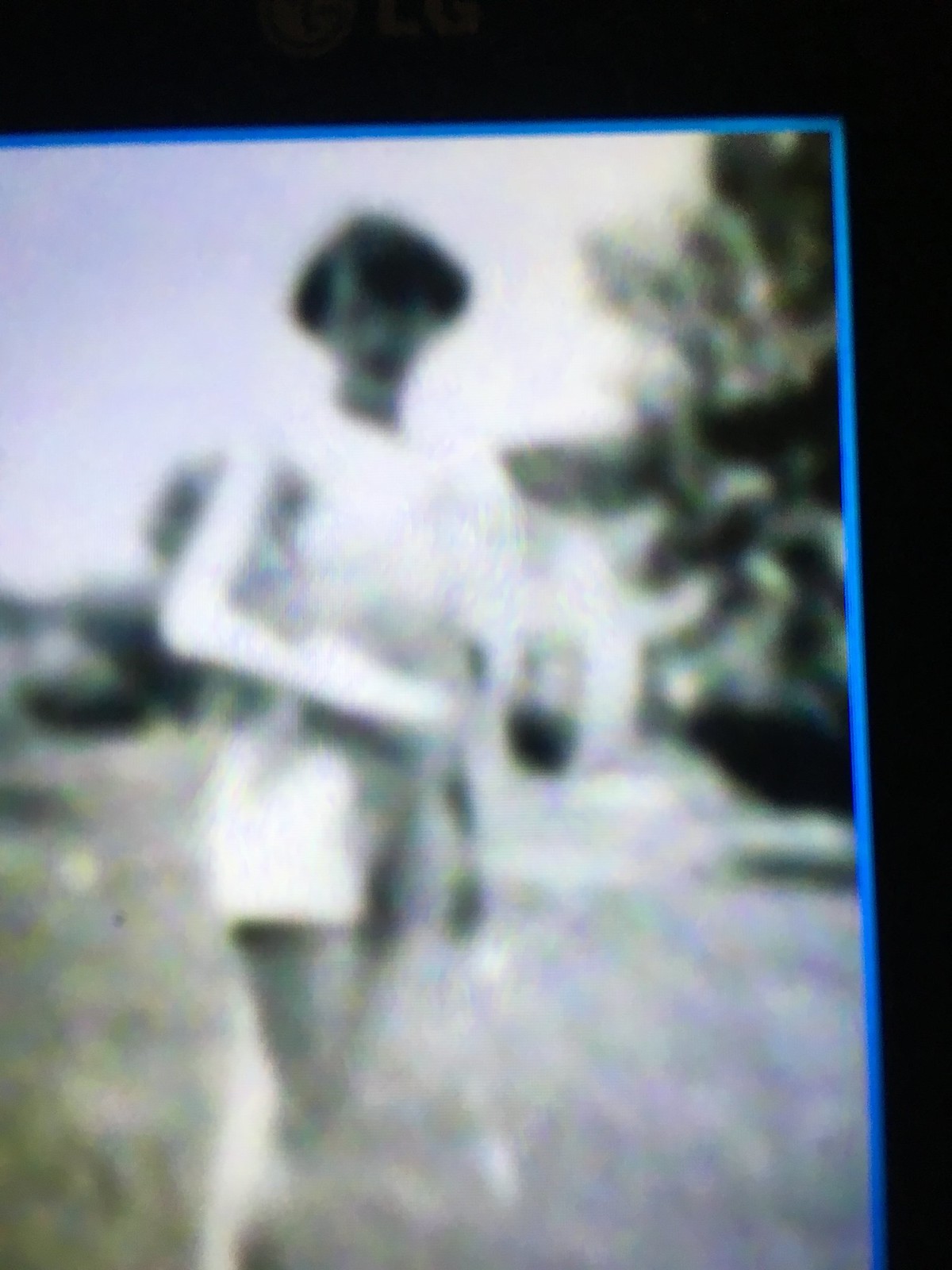In this extremely blurry image, which may itself be a photograph of another photograph, a vintage black and white portrait is featured. The original image appears to date back to the 1940s or 1950s, or perhaps even earlier, capturing a moment from a bygone era. The subject is a woman with short hair, likely black or brown, cropped above her chin. Despite the blurriness, it seems she is wearing lipstick, as her lips appear darker than the rest of her facial features. She is dressed in white shorts, cinched with a black belt, and a white shirt, likely a t-shirt. The photograph ends at her ankles, making her feet unviewable. The entire scene is framed within a blue border, with an additional black border encasing it, suggesting that this might be a photograph taken of the original framed image, possibly using a cell phone.